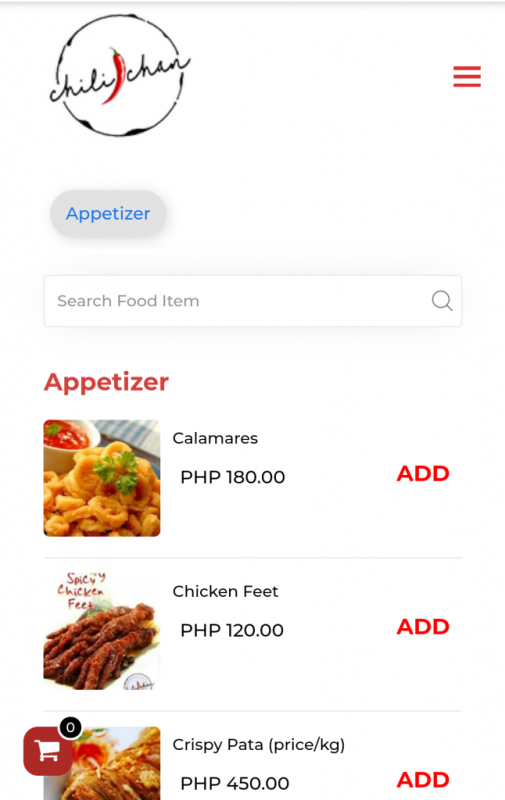The phone screen displays a mobile website featuring the menu of "Chili Chan." The top-left corner shows the restaurant's name elegantly written in cursive within a decorative white circle. The word "Chili" is written first, followed by an image of a red pepper, and then "Chan."

The user has selected the "Appetizer" section of the menu, revealing several items:

1. **Calamari** - Priced at PHP 180.00 with a button labeled "ADD" in bold red letters at the end of the line. There is a small image of calamari on the left side, accompanied by a red dipping sauce.
   
2. **Chicken Feet** - Priced at PHP 120.00, also with a bold red "ADD" button at the end of the line.
   
3. **Crispy Pata** - Priced at PHP 450.00, with the "ADD" button similarly formatted in red.

Each "ADD" button stands out in full capital letters, making it easy for users to add items to their order.